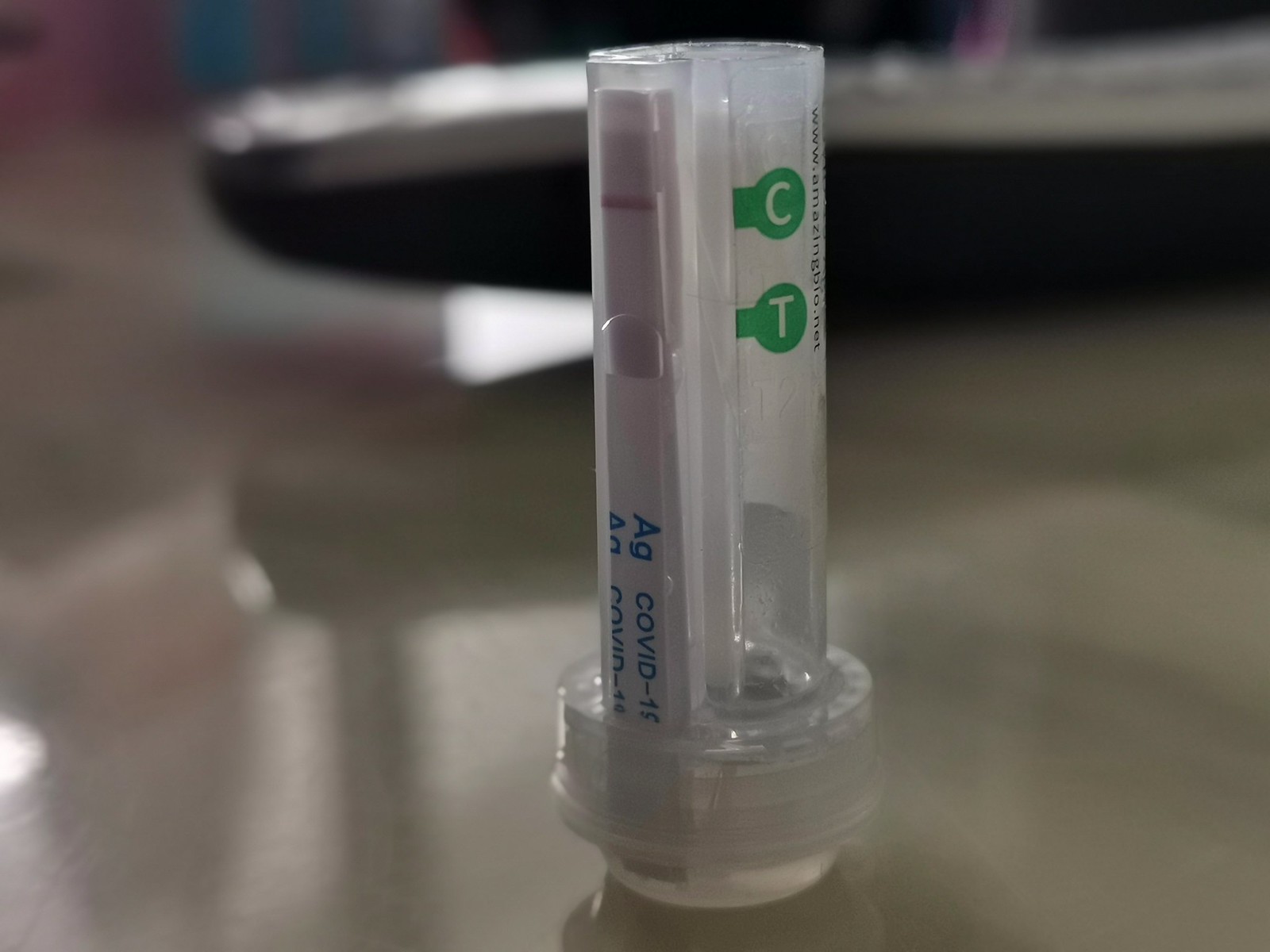In the center of the image is a COVID-19 test kit resting horizontally on a grayish-silver table. The test device, predominantly white with blue lettering, has "COVID-19 AG" clearly marked along its side, signifying it as a rapid antigen test. The result window shows one faint pink line, indicating the test result. To the left of the test is a thick, syringe-like dropper, similar to those used for administering medicine to children. Directly behind the test is an out-of-focus object, appearing black and possibly silver at the top, though indistinct due to the image’s blurriness. The result window on the test also contains the letters "C" and "T" in white capital letters against a green background, with some smaller, unreadable text above it.